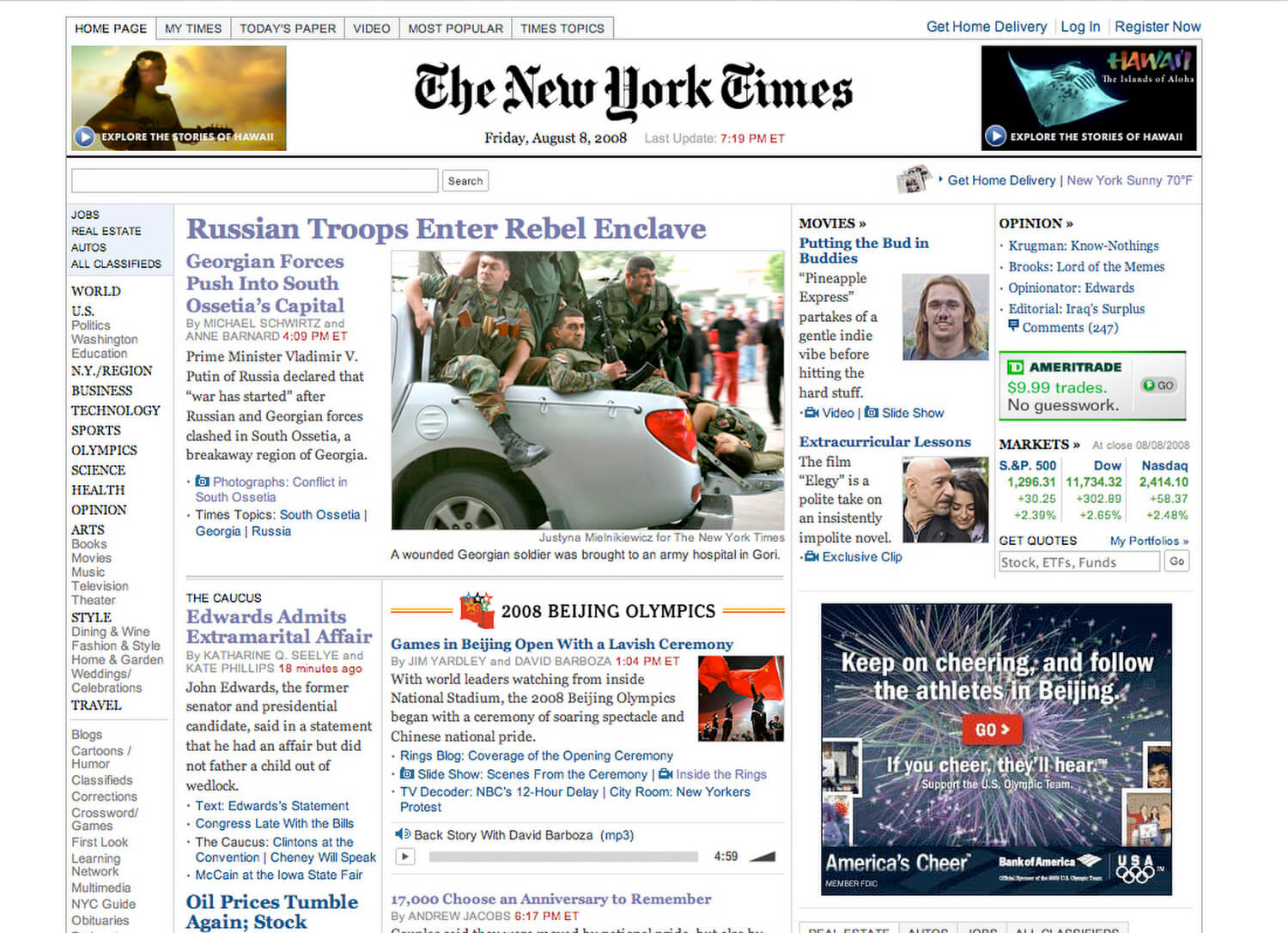This digital edition of The New York Times carries the iconic, classic look and feel of the traditional print version. Dated Friday, August 8, 2008, it features a comprehensive menu bar at the top with options including Page, My Times, Today’s Paper, Video, Most Popular, and Times Topics. The recognizable New York Times calligraphy-style logo is prominently displayed beneath the menu, alongside the date and the latest update time of 7:19 p.m. Eastern.

Flanking the logo are two video advertisements focused on the exploration of Hawaiian stories. Following this, the layout reveals a range of sections, beginning with a left-hand column filled with various categories such as Jobs, Real Estate, Classifieds, Science News, Olympics, Sports, Health News, Art Style and Travel, Comic Section, Crossword Puzzles, TV News, Wedding News, and Dining News.

The main story features a somber photograph of young men dressed in camouflage, sitting in the back of a truck. The image captions a wounded Georgian soldier being brought to an Army hospital in Glory, depicting him lying on his side in evident pain.

Below this main article, there are two additional significant stories. One addresses the conflict in the Caucasus, while another discusses former Senator John Edwards admitting to an extramarital affair. Adjacent to this is a section highlighting the 2008 Beijing Olympics, featuring details about the opening ceremony and a clickable audio clip that provides further information.

To the far right, the page covers movie reviews, such as Pineapple Express and Elegy, alongside stock trade updates and an opinion section. Concluding the page is an advertisement from Bank of America promoting 'America's Cheer,' encouraging viewers to support athletes in Beijing with a link for more information.